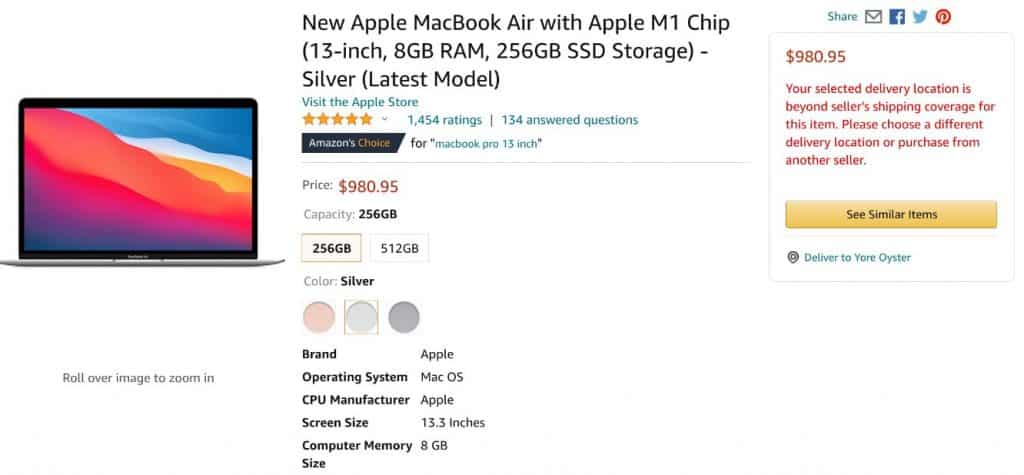**Detailed Caption:**

This is an image captured from Amazon's website showcasing the latest Apple MacBook Air with the new Apple M1 chip. The background of the webpage is a clean white, with a product display taking center stage about two inches over and one inch down from the top edge. The MacBook Air featured has a sleek design with a black border surrounding its screen. The screen's backdrop transitions through various colors starting from a dark blue in the right corner, blending into light blue, then orange, followed by orange-red, purple, and finally gray.

The MacBook Air is supported by a minimalist gray stand directly beneath the screen. About two inches below this setup, there is a small black text prompt that says "Roll over image to zoom in." To the right of this instruction, the product's title is displayed as "New Apple MacBook Air with Apple M1 Chip, 13", indicating the display size. Below that description, additional specifications are listed: "13 inches, 8GB RAM, 256GB SSD Storage." Further down, it specifies "Silver, Latest Model." 

The product details area includes a link to visit the Apple Store, shown in small blue text. The product has garnered significant attention with "1,454 ratings" and boasts a high rating of five stars. Adjacent to this rating, the item is marked with the "Amazon's Choice" badge displayed in dark blue and white, followed by a "New" tag in Amazon's signature yellow.

Pricing details are also provided, revealing a cost of "$980.95" in red text within a small square. Below the price, there are four and a half lines of additional information, accompanied by a yellow tab with black text that says "See similar items." 

On the right-hand side of the page, social media icons for Pinterest, Twitter, Facebook, and email are aligned vertically, followed by a "Share" button. Lastly, there is a location icon next to a blue text reading "Deliver to your location," specifying delivery options.

This comprehensive layout blends detailed product imagery with essential information, helping potential buyers make informed decisions.